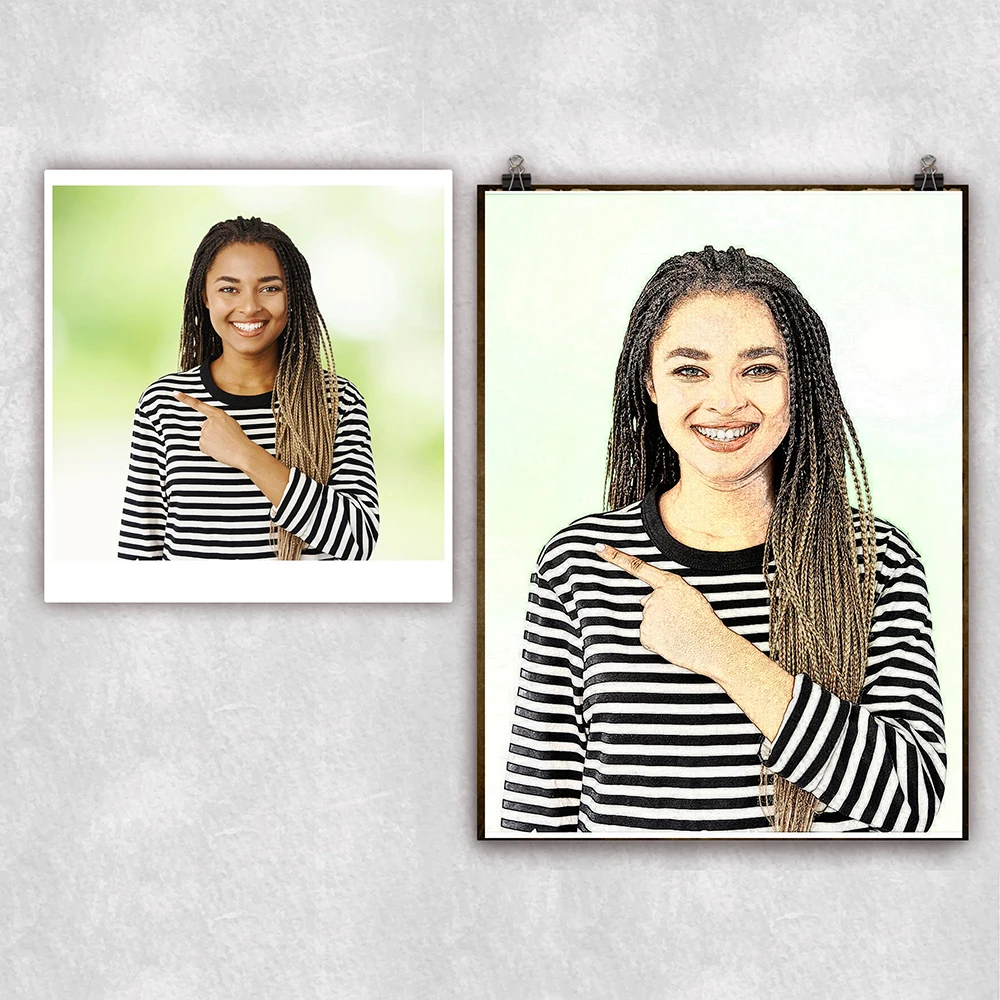The image displays a dual composition featuring a young African-American woman with long braids. On the left side, there is a small, Polaroid-style photograph of the woman, who has brown skin and hair that transitions to a lighter hue at the tips. She is wearing a black and white horizontally striped sweater with a black collar. Her left hand is raised, pointing to the upper left corner, and she smiles engagingly at the viewer, displaying pink blush lipstick and white teeth. The background of the photograph consists of green and white blurred blobs. This image is framed by a white border. 

On the right side is a larger colored pencil illustration that faithfully replicates the photograph. The illustration portrays the woman in the same pose and attire, with careful attention to her long braids and expressive smile. The two images are set against a gray paper background, giving the impression that the illustration is a stylized rendering of the original photograph. This juxtaposition highlights the contrast between the photographic realism and the hand-drawn artistic interpretation.